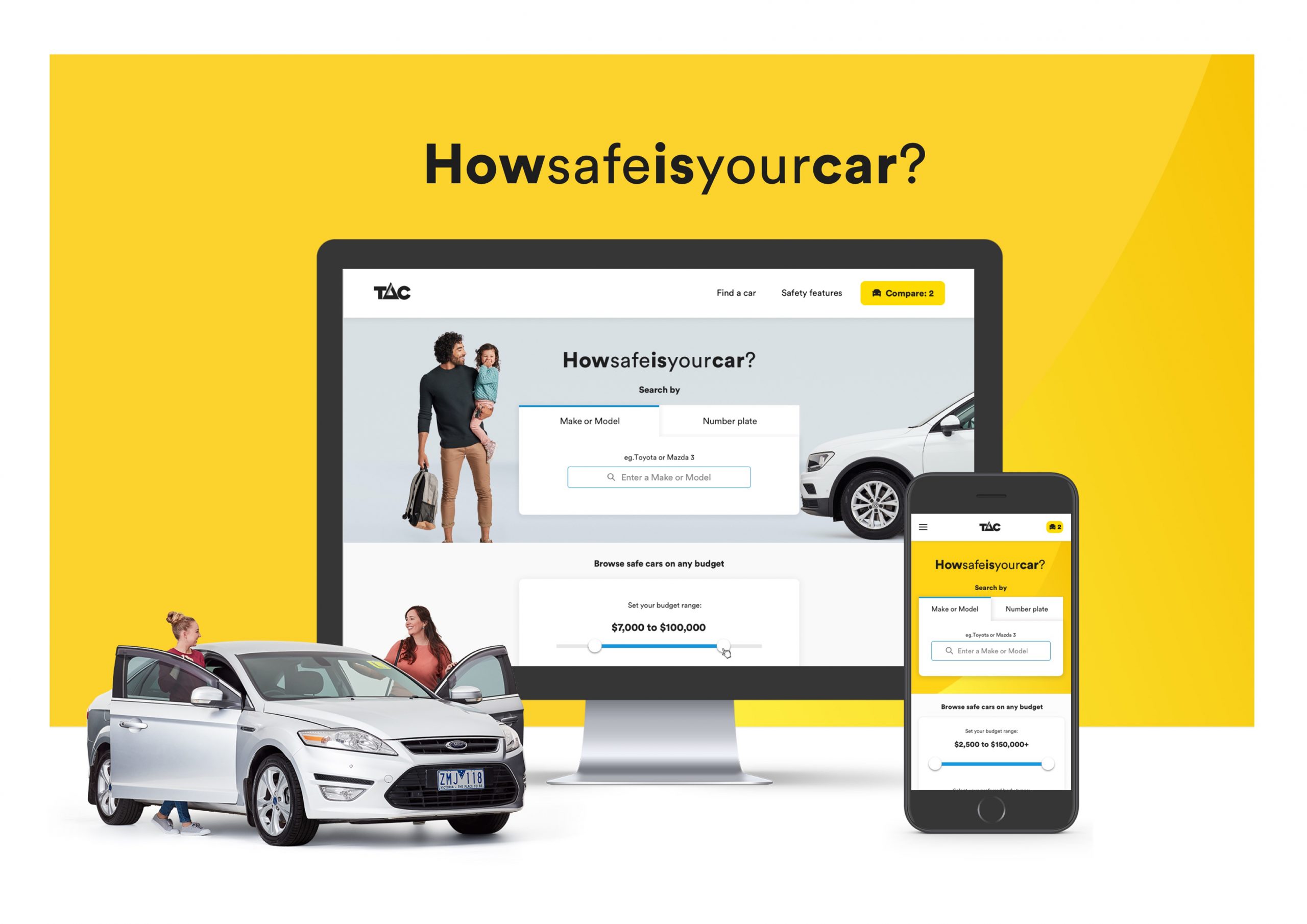This image features a screenshot from a webpage titled "How Safe Is Your Car." The central section of the screen showcases a Mac displaying a website with an interactive car safety information page. On the screen, a man is shown holding his child while standing beside his car, emphasizing family safety.

The webpage includes a variety of interactive elements and text, such as "Find a Car," "Safety Features," "Compare," and "Search by Make or Model." There is also a search field at the bottom, offering examples like "Toyota" or "Mazda 3," and options to browse cars by budget, from $7,000 to $100,000.

Accompanying this, an iPhone is depicted, showing a similar interface with a price filter range from $2,500 to $850,000. The phone interface also displays choices for car colors, listing black, silver, white, and yellow.

Two women are positioned at each of the front doors of a vehicle, facing each other, adding a human element to the scene. The image effectively combines elements of technology and personal interaction, emphasizing ease of access to car safety information.